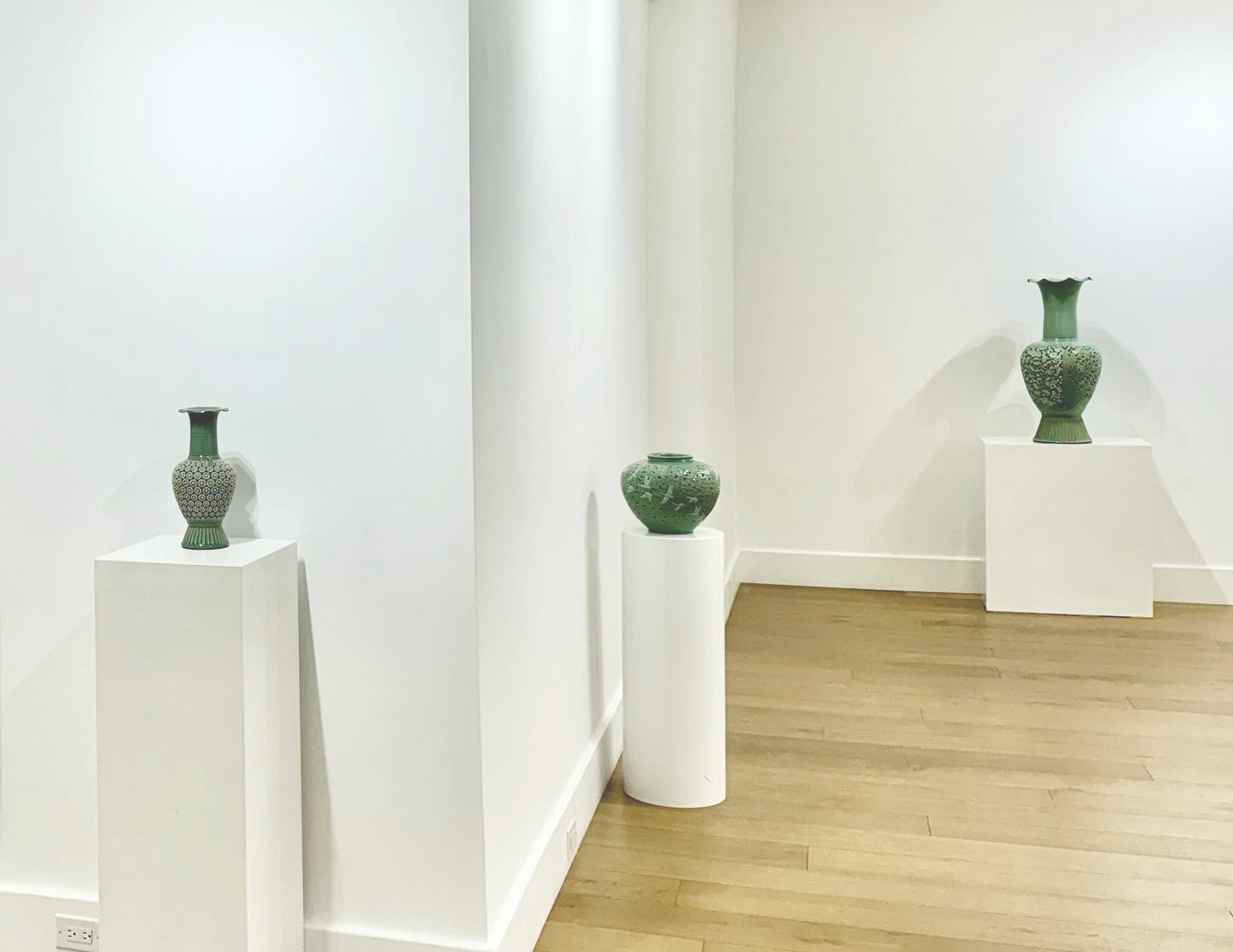This photograph captures an angled view of a minimalist art gallery featuring pottery on display. The gallery is characterized by its bright white walls and white woodwork trim at the base, complemented by light tan wood flooring. The pottery, all in a light jade green hue with delicate white accents and intricate indentations, is elegantly presented on pedestals of various shapes. 

To the left, a tall rectangular white pedestal showcases a slim vase with a long neck and a wide base. Around the corner, a cylindrical white pillar supports a more rounded vase, distinguished by its rounded opening and balanced proportions. To the right, against a third wall, stands a square pedestal with a large, prominent vase that features a broad base, a substantial center, and an elongated neck. Each piece varies in size and shape, enhancing the aesthetic diversity of this serene and carefully curated gallery space.